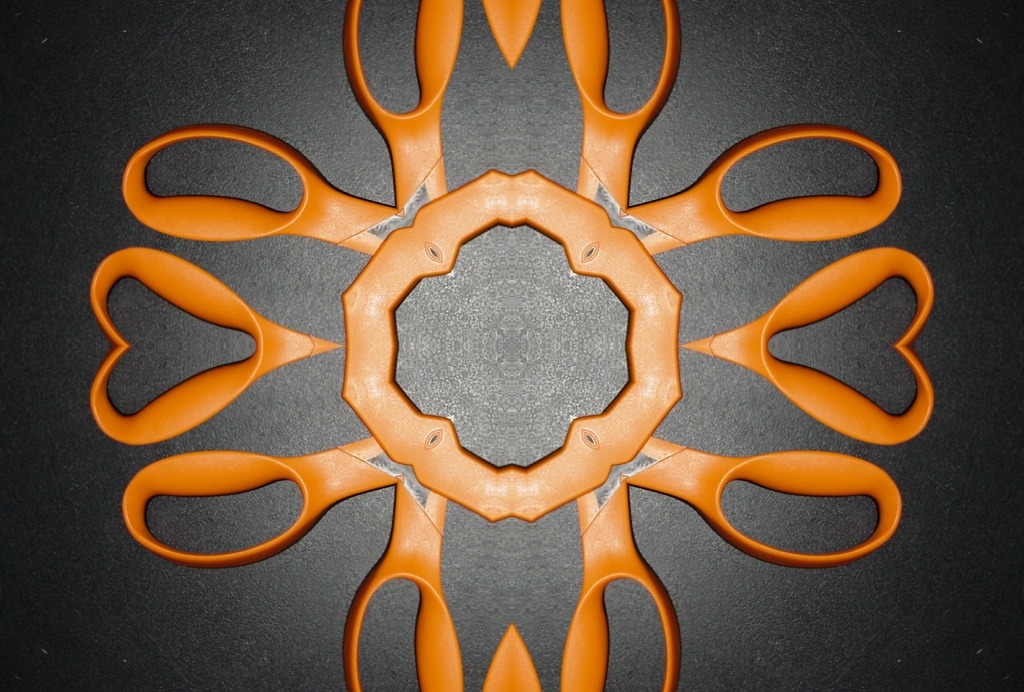The image showcases a striking sculpture made predominantly from the handles of orange scissors, intricately arranged into a detailed, flower-like design. The handles, some of which are cut or melted, radiate outward from a central point, creating heart-shaped formations on the periphery and forming a diamond-like shape in the center. This central area, composed of melted plastic from the scissors, resembles a flower's core and is accentuated by a black platform with light illuminating it. The entire arrangement sits on a gray, intricately designed surface, emphasizing the aesthetic cohesion of the piece. This art piece, possibly involving 9 pairs of handles, merges the industrial with the artistic, transforming everyday objects into a unified, visually captivating sculpture.